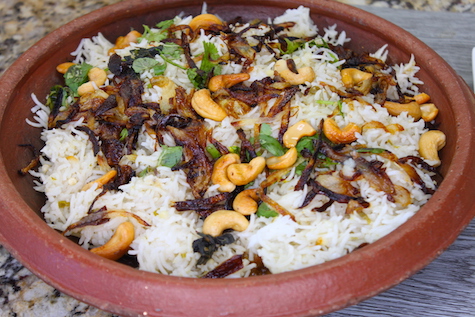The image depicts a close-up photograph of a bowl of food prominently placed on a wooden table, sitting atop what seems to be a wooden palette. The bowl, which has a dark reddish-brown or terracotta-like color with a rough texture, features high brims and a round shape. Inside the bowl, there's a plentiful serving of white basmati rice. Scattered and mixed with the rice are large, curved nuts that resemble almonds or pistachios. The dish also contains dark, caramelized onions that have a crispy, sautéed appearance. Interspersed among the rice and nuts are sparse, dark green leaves, possibly green peppers or plant leaves, adding a hint of color to the predominantly white and brown dish. The rice, nuts, and caramelized onions together give the impression of a flavorful, possibly Asian-inspired culinary creation.